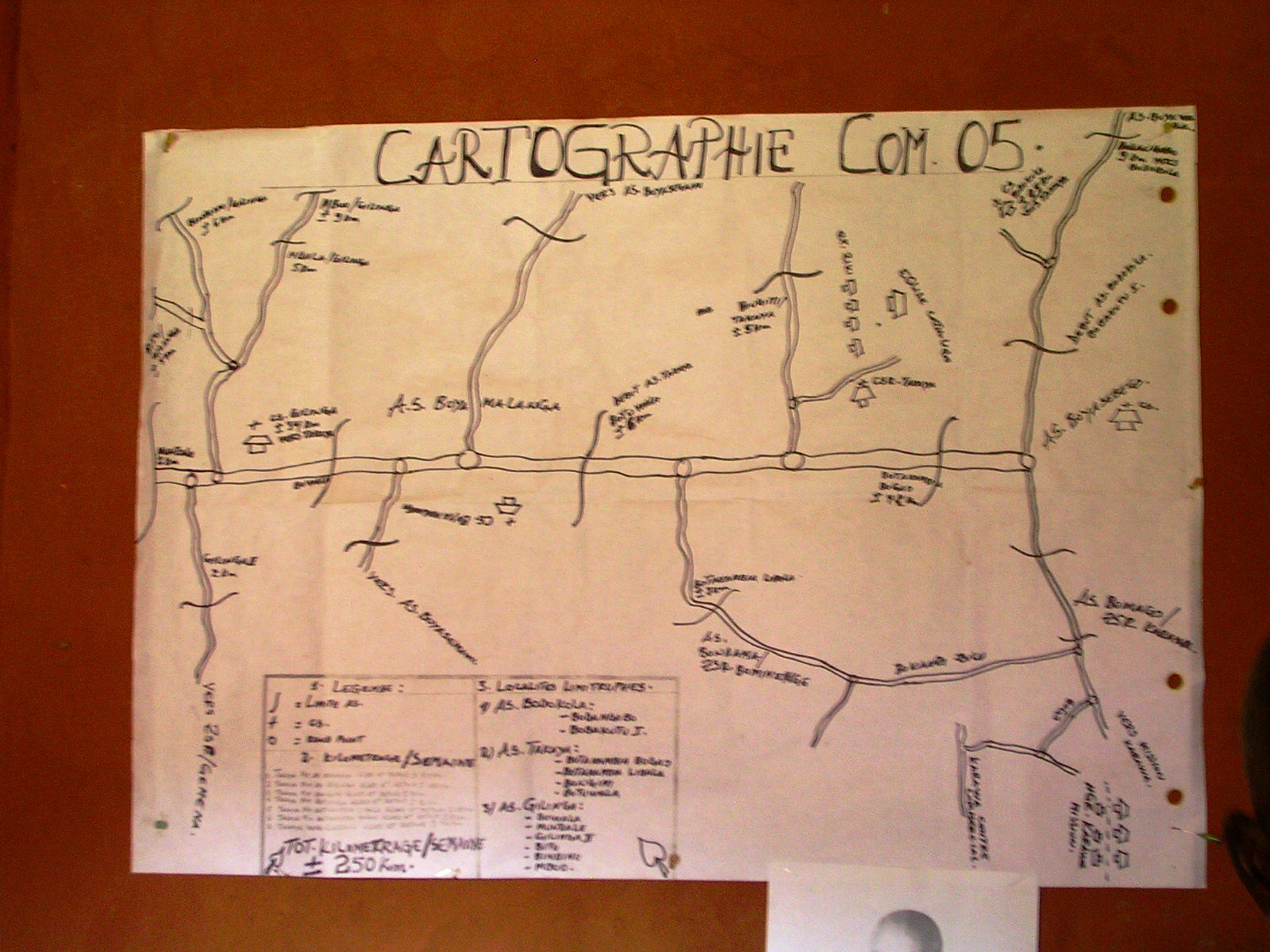The photograph depicts a hand-drawn, wrinkled map labeled "cartography COM 05" at the top. The map appears to be on a brown wall and shows a central main path with numerous tributary-like lines extending from it. Each place on the map is marked with small, handwritten text that is difficult to read. In the bottom left corner, there's a detailed legend explaining the symbols used throughout the map. Towards the bottom right, partially covering the map, a picture with a gray circle tacked over appears. The map's overall presentation suggests it has been frequently handled and folded, revealing a complex network of paths and symbols.